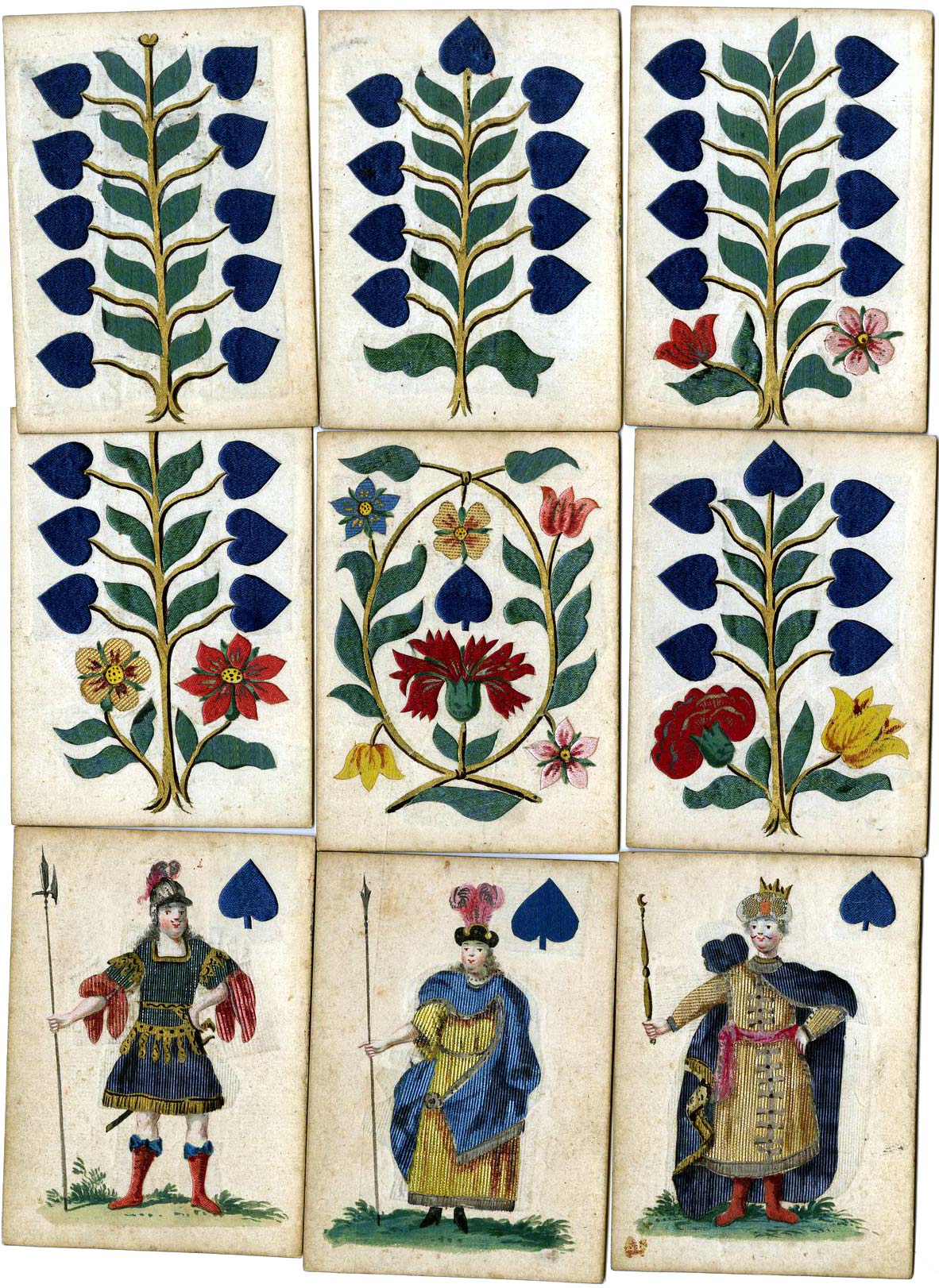The image showcases nine old-fashioned playing cards arranged in a 3x3 grid. The top two rows display various trees, leaves, and flowers, with the first row primarily featuring leaves and the rightmost card adorned with two flowers, one red and one pink. The middle row combines flowers with leaves. The bottom row is dedicated to royalty, depicting characters in elaborate, period-specific attire. One card features a regal man in a helmet, billowing sleeves, a skirt, calf-high shoes, holding a sword and staff. Another card portrays a crowned woman in a dress, wielding a staff. The final royal card shows a man in a dark cape, red sash, red boots, and a crown, holding a shorter staff. All the cards have a weathered, antique look, reminiscent of designs from the 1500s.